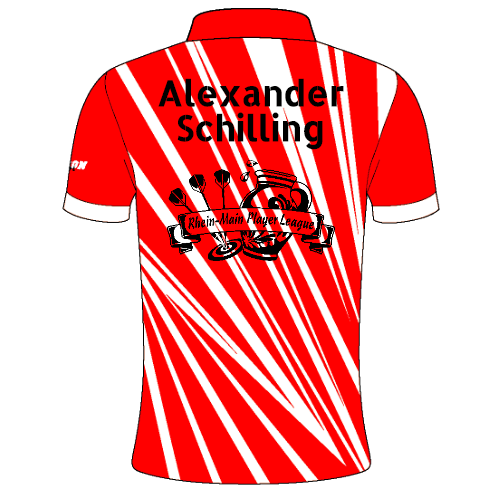The image is a highly detailed color drawing of the back of a red football kit, prominently set against a plain white background. The kit features an intricate design of white stripes in varying sizes that run diagonally across the red base. Both short sleeves of the kit are edged in white, with one sleeve displaying a few small, unreadable white letters. The back of the kit is adorned with black text; at the top, it reads "Alexander Schilling" in bold letters. Below this name is a banner that says "Rhyne Main Player League." Situated beneath the text is an illustrative element – a bullseye with three darts precisely lodged in the center and an image of a pitcher. This composition suggests an advertisement-like quality, reminiscent of promotional material for a sports team or league.